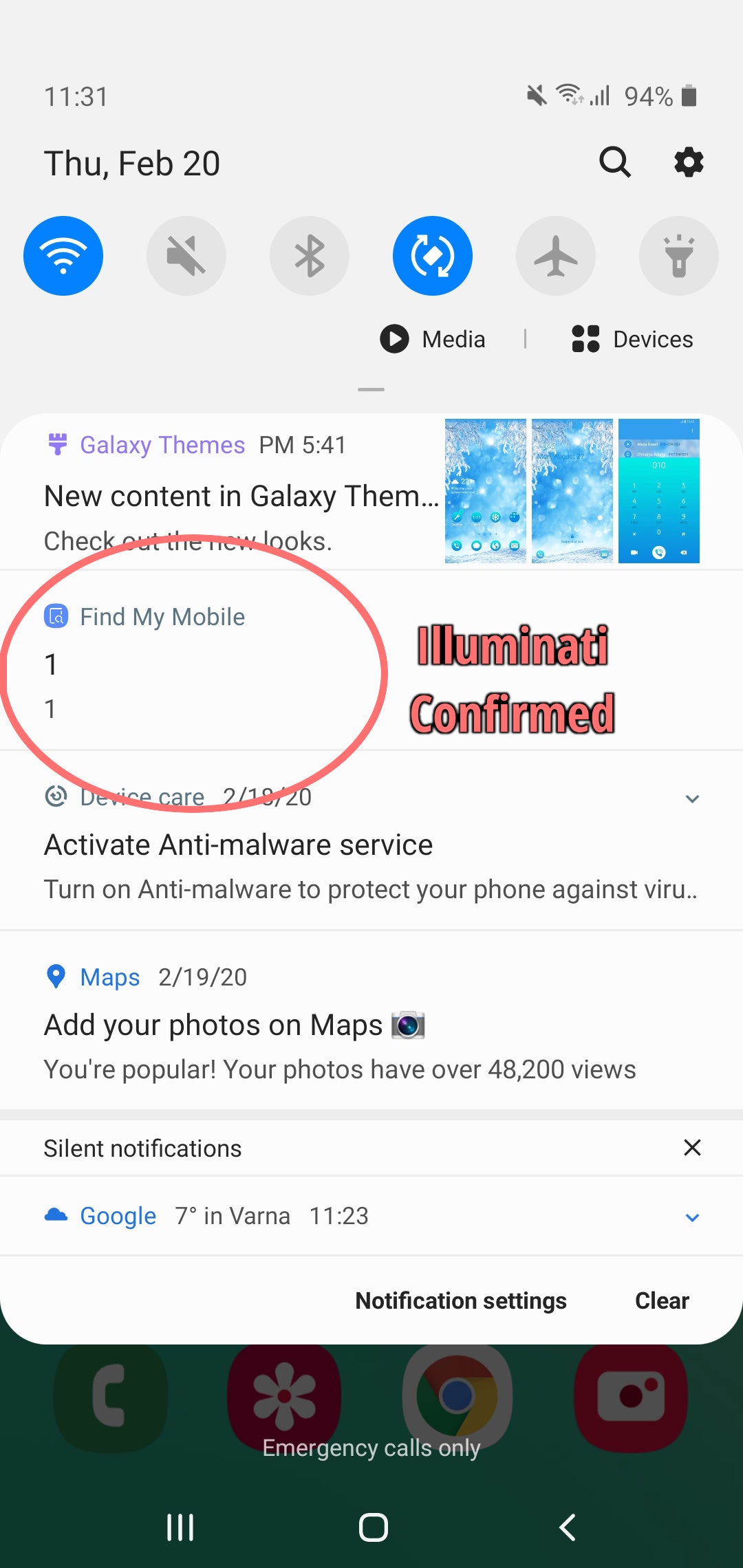**Caption:**

A detailed screenshot captured from a mobile phone showcases various on-screen elements:

- **Top Bar Details:** 
  * Time displayed is "11:31" at the top left corner.
  * To the right are icons: a muted sound button, a filled Wi-Fi icon, a filled signal strength icon, "94%" battery level, and nearly fully charged battery icon with a thin white line indicating remaining capacity.

- **Mid Section Information:**
  * Date shown on the left as "Thursday, February 20th."
  * To the right, a magnifying glass icon (search) is followed by a cogwheel icon (settings).

- **Wi-Fi Status:**
  * Below the date, a blue-filled Wi-Fi icon in a circle on the left, with adjacent settings-related icons.

- **Media and Devices Section:**
  * The next line specifies "Media" with a play button icon, separated by a line, and "Devices" to the right.

- **Galaxy Themes Notification:**
  * Displays "Galaxy themes" with a note about new content, although ‘theme’ is cut off partially.

- **Find My Mobile & Notifications:**
  * A red circled "Find My Mobile" notification, followed by "11" encircled and the text "Illuminati confirmed."
  * Instructions to "activate anti-malware service," albeit cut off, and "add your phone on Maps."

- **Silent Notifications:** 
  * Mentions "silent notifications" with a Google icon paired with a cloud sign.
  * Temperature information at "7 degrees in Verna, 11:23."

- **Bottom Options:**
  * At the bottom, options to adjust "notification settings" or "clear all notifications."

This comprehensive detail captures the essence and specific content visible in each segment of the screenshot.